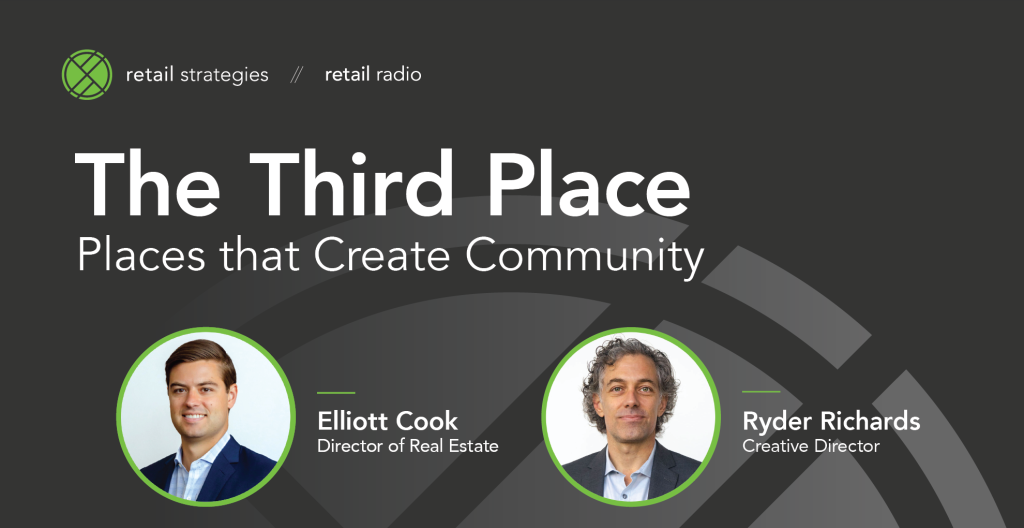The image appears to be a digital title screen, likely from a company's web page or a PowerPoint presentation introducing two key figures from the organization. The background is dark gray, featuring a faint, larger version of a green circular logo with a diagonal line intersected by two equal signs.

At the top left, next to the green logo, the text "Retail Strategies" is displayed in white, followed by a divider, and then "Retail Radio" also in white. Below this, in the largest font, it reads "The Third Place," with the subtitle "Places That Create Community" in smaller, non-bold text. 

Underneath this heading are two photographs framed by green circular outlines. The first, on the left, pictures Elliot Cook, a European man with brown hair, wearing a blue suit jacket and a light blue collared shirt. His name is displayed in bold white text with a green line above it, and beneath his name, the title "Director of Real Estate" is in non-bold text.

To the right is another man, aged and of European descent, with curly dark brown and gray hair. He is clad in a dark blue or black blazer and a light blue collared shirt. Above his bold white name "Ryder Richards" is a green line, and below it, his title "Creative Director" is in non-bold text. Both men are presented against the same dark gray background, lending uniformity to the slide.